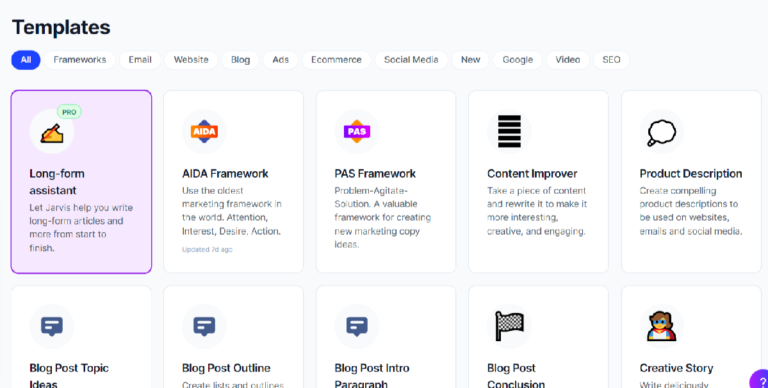**Image Description:**

The image features a user interface on a grey background. In the upper right-hand corner, the word "Templates" is prominently displayed in black font. Below this title are a series of clickable category buttons with oval shapes, organized horizontally. The first button reads "All" and is highlighted in blue with white font, signifying it is the selected category. The other category buttons, each in white with grey font, include "Frameworks," "Email," "Website," "Blog," "Ads," "E-commerce," "Social Media," "New," "Google," "Video," and "SEO."

Under the category buttons, some categories are loaded into white rectangular shapes showcasing different templates. Detailed descriptions for each template are displayed as follows:

1. **Long Form Assistant**: "Let Jarvis help you write long form articles and more from start to finish." This selection is highlighted with a purple box around it.
2. **AIDA Framework**: "Use the oldest marketing framework in the world. Attention, Interest, Desire, Action."
3. **PAS Framework**: "Problem and Solution. A valuable framework for creating new marketing copy ideas."
4. **Content Improver**: "Take your piece of content and rewrite it to make it more interesting, creative, and engaging."
5. **Product Description**: "Create compelling product descriptions to be used on websites, emails, social media."

At the bottom of the display, partially visible template categories include "Blog Post Topic Ideas," "Blog Post Outline," "Blog Post Intro Paragraph," "Blog Post Conclusion," and "Creative Story."

The focus of the interface, indicated by a highlighted purple box, is currently on the "Long Form Assistant" template.